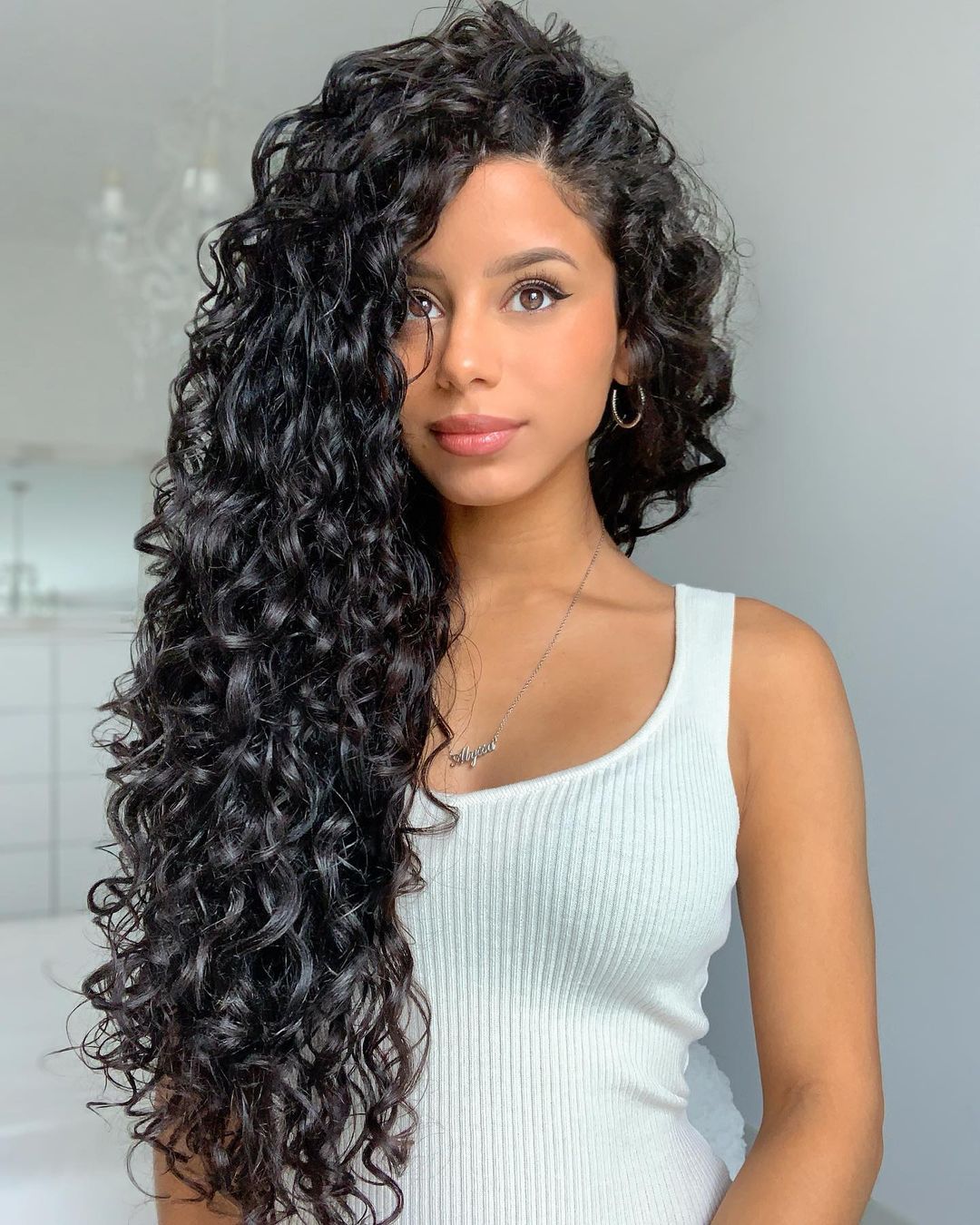A photograph of a beautiful young woman with very long, curly dark hair cascading down around her right shoulder, partially obscuring the right side of her face and body. She has a medium to dark complexion, full pink lips, and dark brown eyes. She is wearing a white tank top that contrasts elegantly with her skin tone. Her makeup is subtle but noticeable, with a hint of red lipstick highlighting her lips. The woman is adorned with a silver necklace bearing an emblem with script writing, and a single earring is visible on her left ear while her right ear is covered by her flowing hair.

The background is a softly out-of-focus white interior, possibly a bathroom or bedroom, suggesting wire racks and drawers, and featuring a blurred chandelier hanging above. The indoor setting and blurred backdrop ensure that the emphasis remains entirely on the young woman, who stands upright, gazing directly at the camera in what appears to be a modeling photo. The image captures her from the top of her head to just above her waist, framed in a vertical rectangle. The color palette of the photo features a mix of black, white, tan, pink, brown, gray, peach, beige, and silver, emphasizing the natural and serene mood of the portrait.